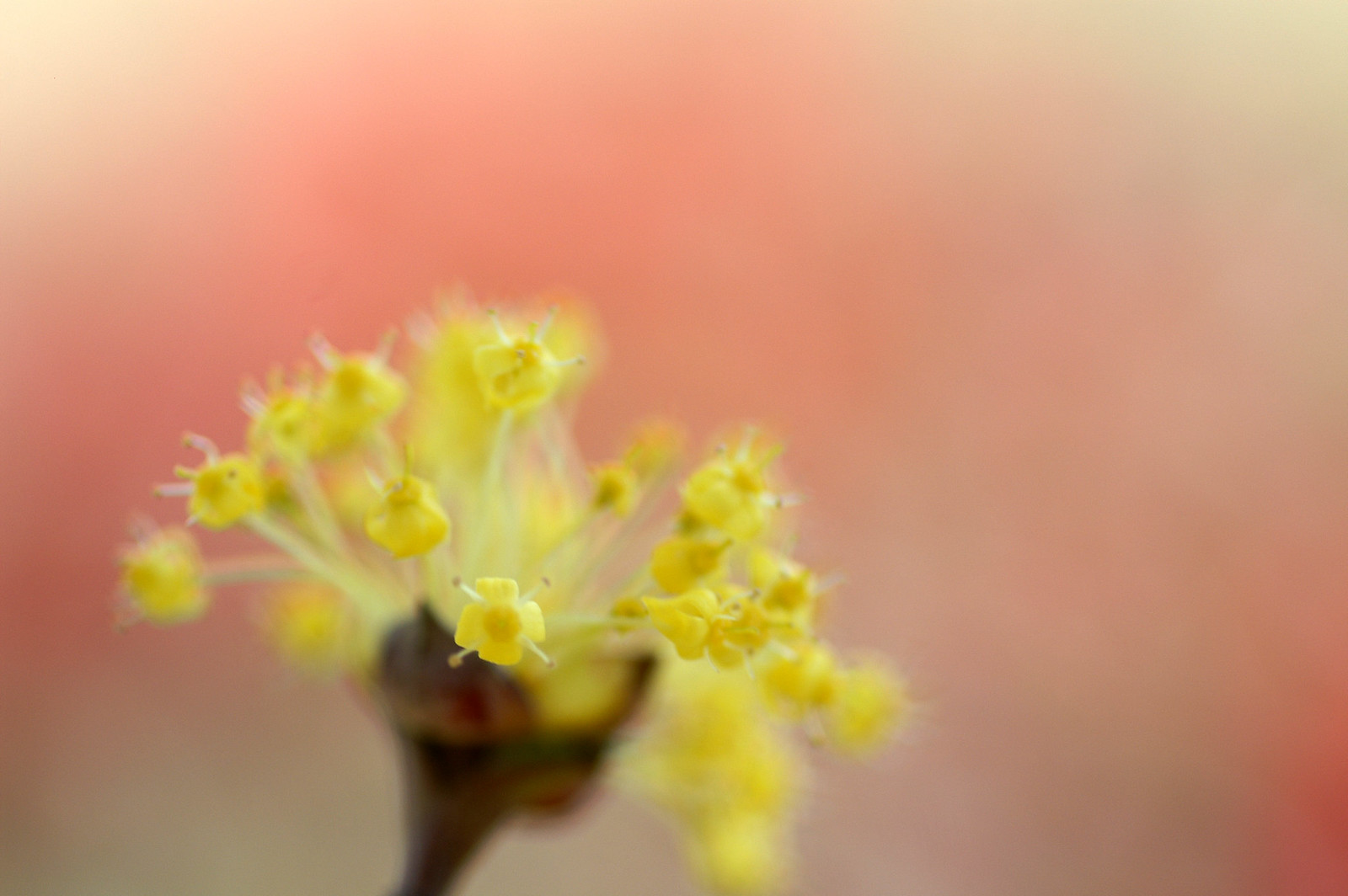The image is a rectangular photograph capturing a delicate and peaceful scene with a single, prominent flower slightly off-center towards the bottom left. The flower is depicted with intricate detail, displaying a brownish base from which multiple yellow shoots sprout. These shoots are adorned with small, white stems that culminate in tiny yellow flowers, each with four petals and a darker yellow center. The flower's stem exhibits a mix of browns, yellows, reds, and greens, adding to the complexity and beauty of the image.

The background is an indistinct blend of colors, predominantly pinks, oranges, and creams, creating a soft, serene ambiance. The photograph is imbued with natural light, suggesting it might have been taken outdoors or in a well-lit indoor space. Despite the blurry background, the vibrant colors seamlessly merge into each other without forming any discernible shapes, emphasizing the tranquil vibe. The composition effectively highlights the intricate details of the bloom against the soothing, pastel hues of the backdrop.